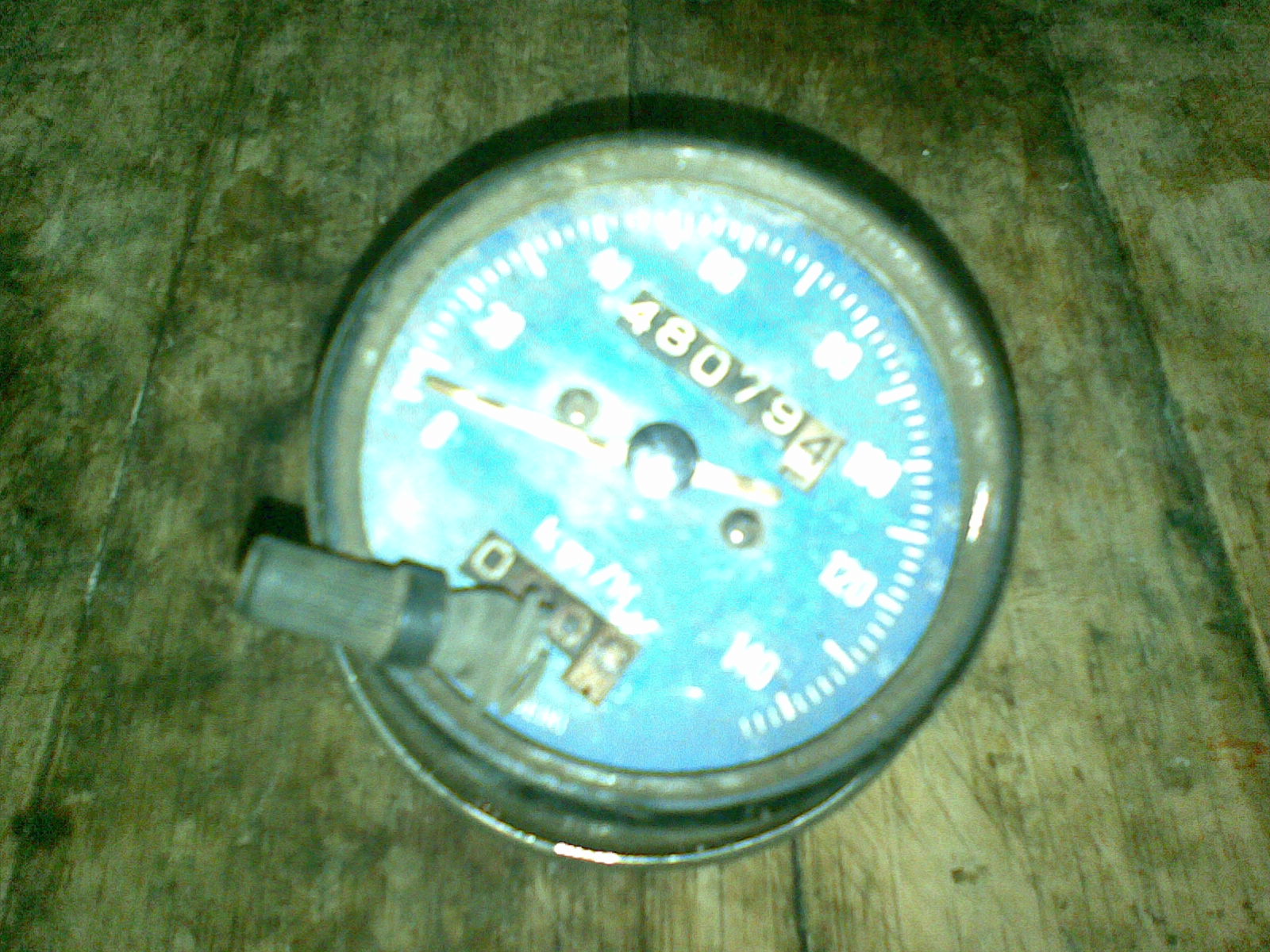A detailed close-up of an unmounted, slightly dirty, blue-faced meter resting on a wooden surface. The meter, which appears to be slightly rusted, features a metallic rim encircling its dial. The dial ranges from 0 to 140, marked in increments of 20, with the number 480794 displayed prominently. A small pipe extends from one side of the meter but is not connected to any apparatus. The bright lighting overexposes some areas of the image, making it challenging to identify further details.